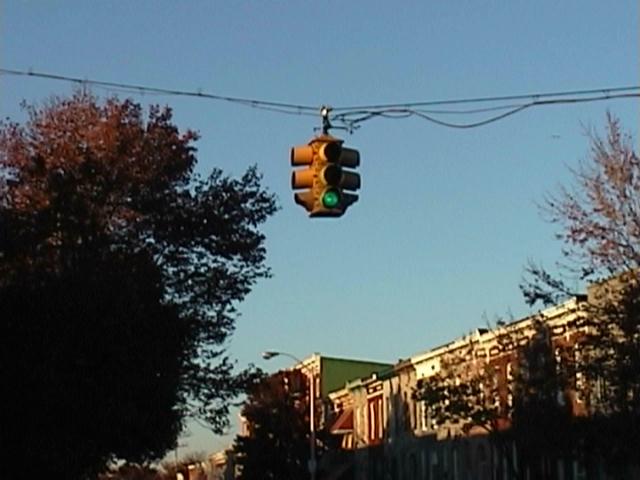In this image, a traffic light is conspicuously suspended in mid-air by a black cable running horizontally across the top portion of the scene. The traffic light is illuminated green, with additional lights facing left and right, although their current states are not visible. The backdrop features a clear, bright blue sky devoid of any clouds. On the left side of the image, a large tree adorned with reddish leaves suggests an autumnal setting. To the right, a series of storefronts stretch diagonally into the distance. These buildings share a cohesive color palette, predominantly featuring shades of red, light brown, and beige, which harmonize with each other. A prominent streetlight is present, and further back stands a taller green building, partially obscured by additional trees. The overall scene has a slightly blurred quality, yet the key elements remain discernible, painting a vivid picture of a bustling urban environment in the fall.